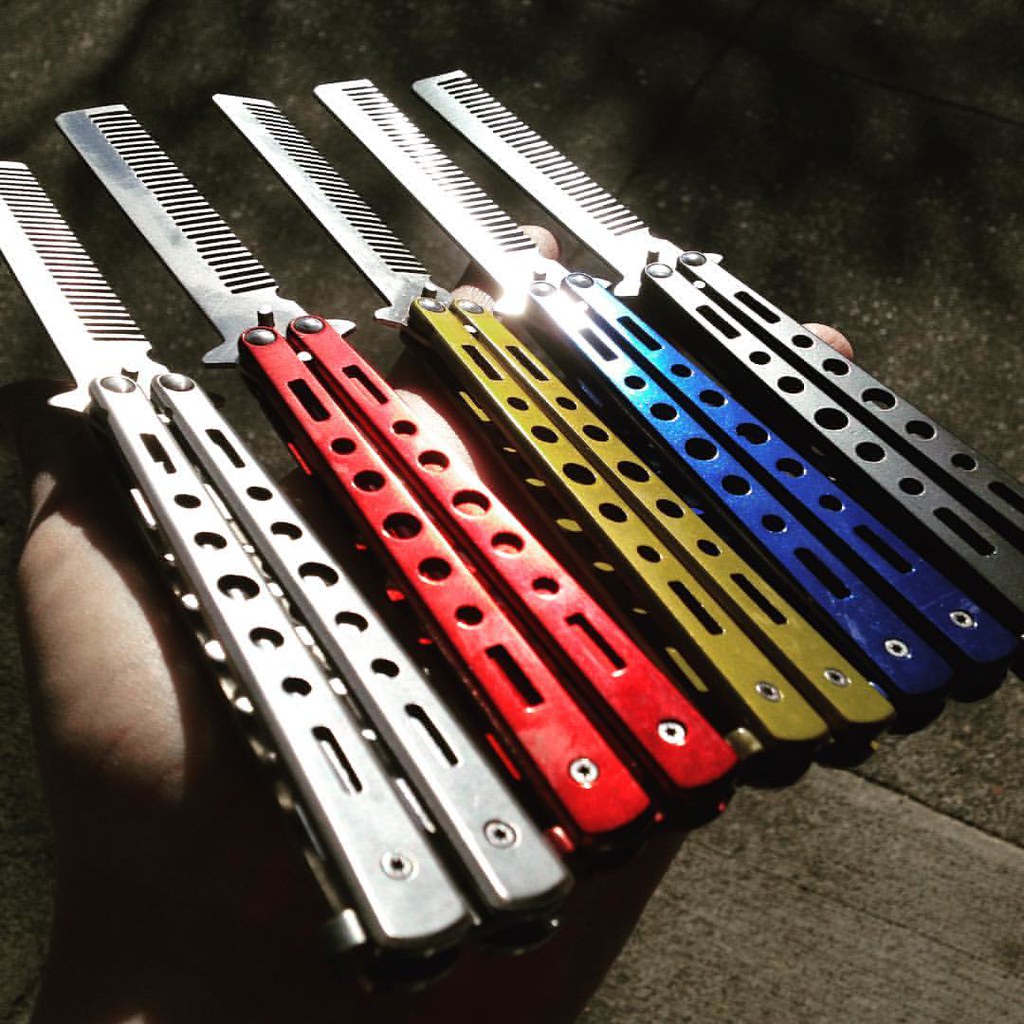This photograph captures five switchblade-style combs, each featuring distinctively colored metallic handles with several circular holes and additional rounded rectangular holes at both ends. The comb handles, reminiscent of multi-tool designs, come in a sequence of colors: silver, red, gold, blue, and a darker silver. Each comb is in an open position with the teeth all uniformly facing to the right, and all comb parts have a reflective silver finish, capturing the light subtly. The combs are resting flat on a person's upward-facing palm, a hand which is only partially visible. The background comprises a cement surface divided into two shades, with a darker gray on the upper portion and a lighter shade at the bottom, providing a contrasting backdrop to the vibrant handles of the combs.